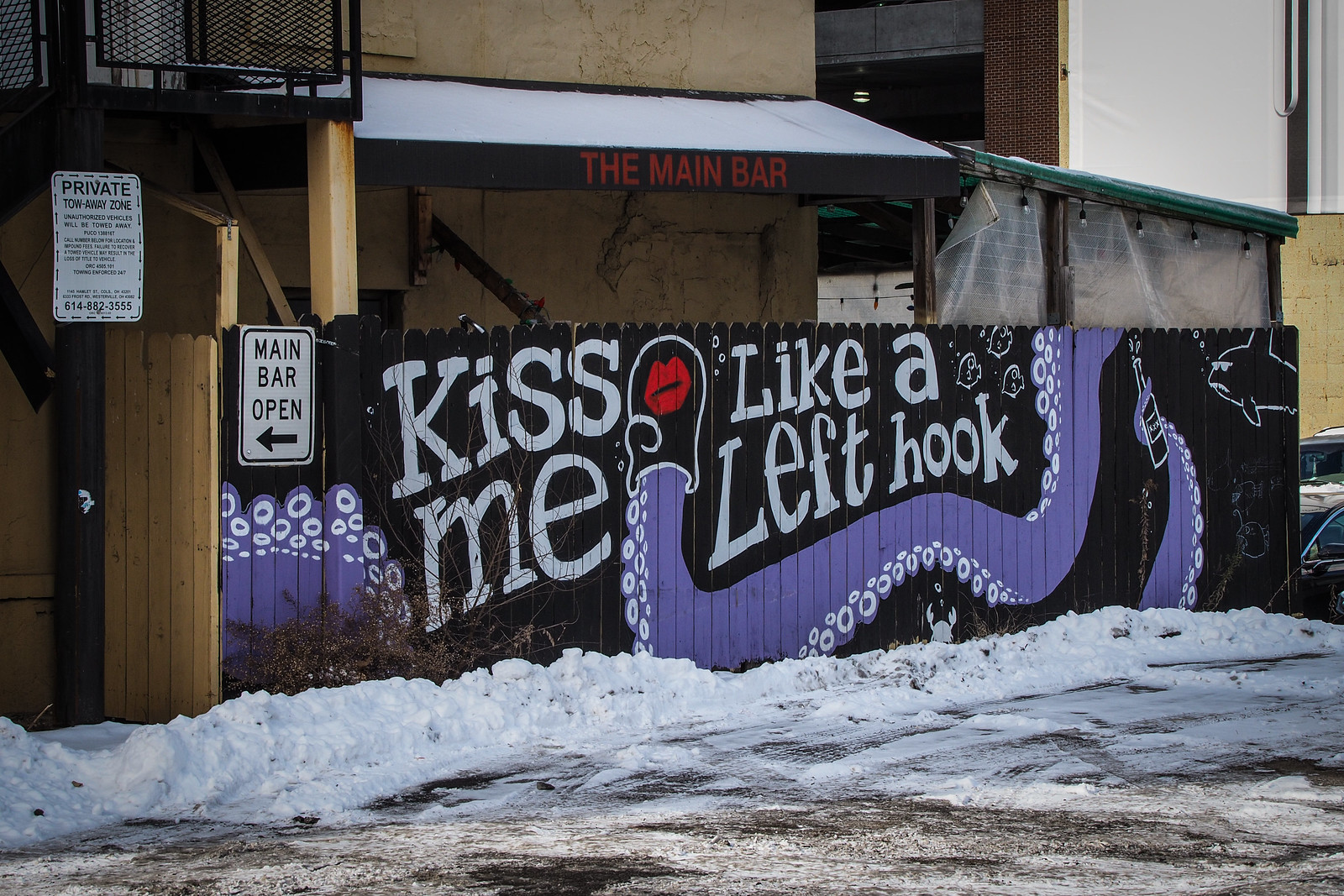The image depicts a wintery scene outside a bar named "The Main Bar." The ground is covered in snow, indicating it is wintertime. Prominently featured is a dark brown fence adorned with detailed and vibrant artwork. The focal point of the art is a purple octopus tentacle, which stretches across the fence. This tentacle is holding a bottle of alcohol and has red lips near the tip, framing the painted words "Kiss me like a left hook." Enhancing the quirky artwork, a fish with a mustache and glasses is depicted on one side. On the left side of the fence, a sign with white letters on a black background reads, "Main Bar Open," pointing towards a plain wood fence door. Above the door, another sign indicates a "Private Tow Away Zone," suggesting this is part of a parking lot or back alleyway.